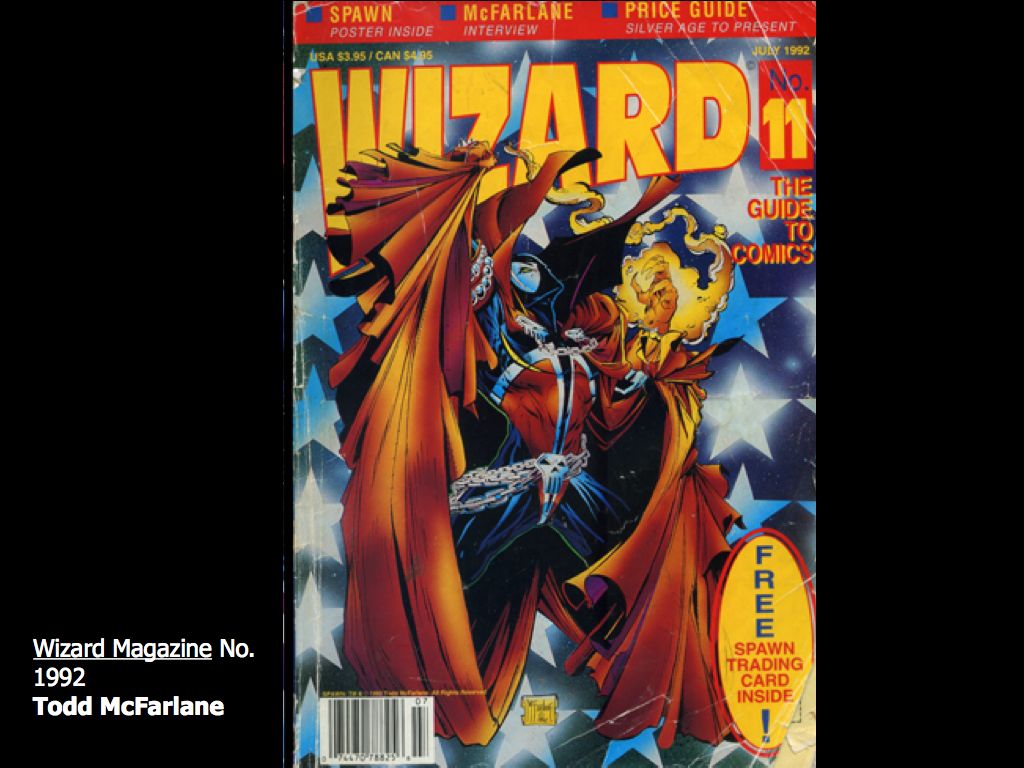The comic book cover features the bold, blocky yellow title "Wizard" prominently displayed across the top. Dominating the center is a vividly colorful image, primarily in shades of reddish-yellow, depicting large wings that seem to envelop a darkish-gray-blue wizard. The wizard, who might also be situated in a cave, boasts a skull ornament attached to a chain wrapped around his waist. His chest is adorned with striking red and white colors, while his dark hood shadows his pale face. The background is adorned with a scattering of blue and white stars, adding to the mystical atmosphere. Above the wizard, the words "Spawn," "McFarlane," and "Prize Guide" are featured prominently. In the bottom left corner, the text "Wizard Magazine, No. 1992, Todd McFarlane," is printed in white, detailing the issue and contributing artist.